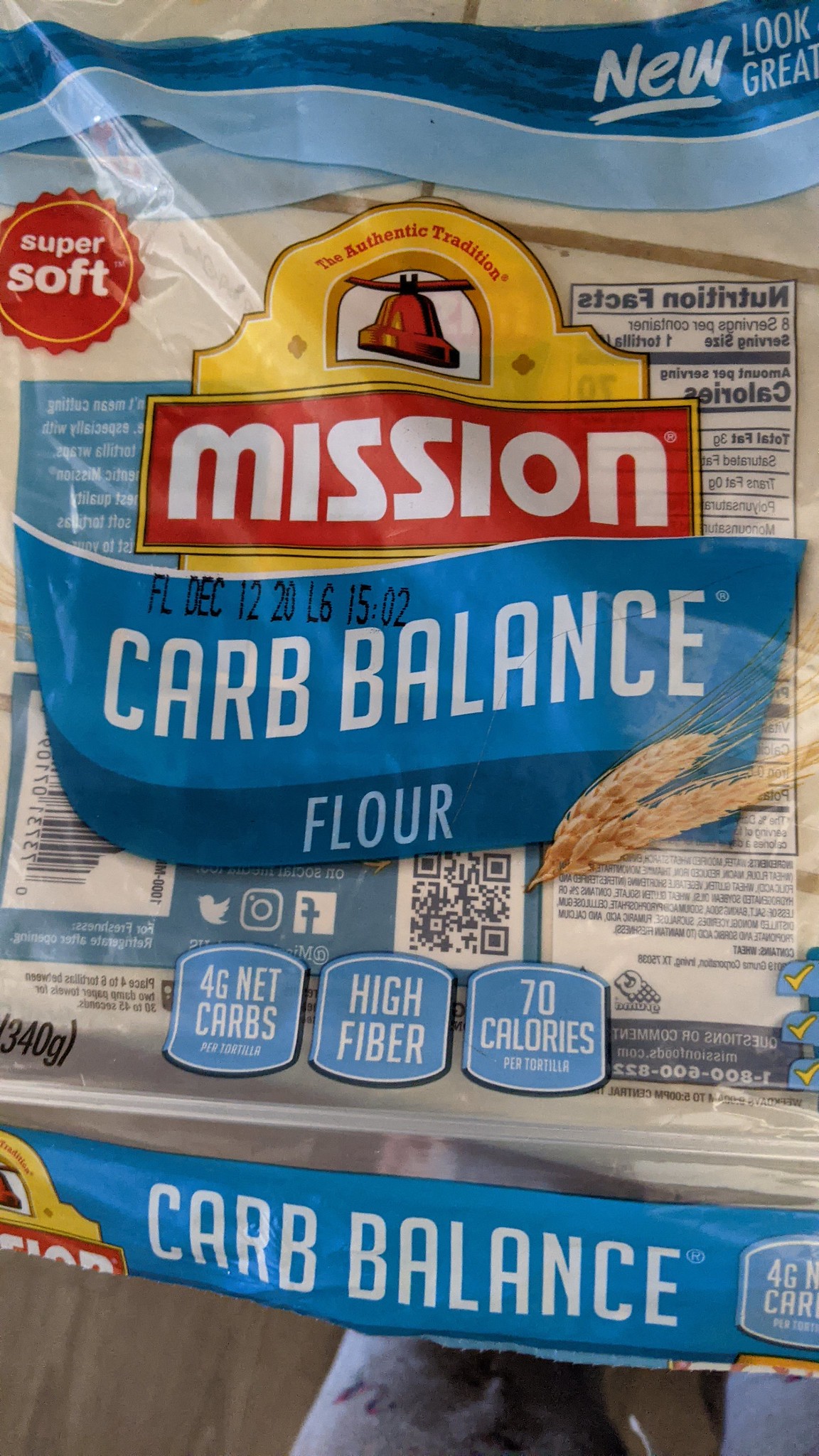This is a packet of "Mission Carb Balance Flour" tortillas, boasting the tagline "Super Soft New Look Great The Authentic Tradition." The packaging, semi-transparent in parts, prominently features blue banners and a depiction of a wheat head, signifying its flour content. The design includes muted red and yellow accents, giving the packaging a subdued appearance. Key nutritional highlights are prominently displayed in blue, rounded squares with white font, proclaiming 4 grams net carbs, high fiber content, and 70 calories per serving. The back of the packet, which is also semi-transparent, reveals additional nutritional information, creating a somewhat cluttered but informative presentation.